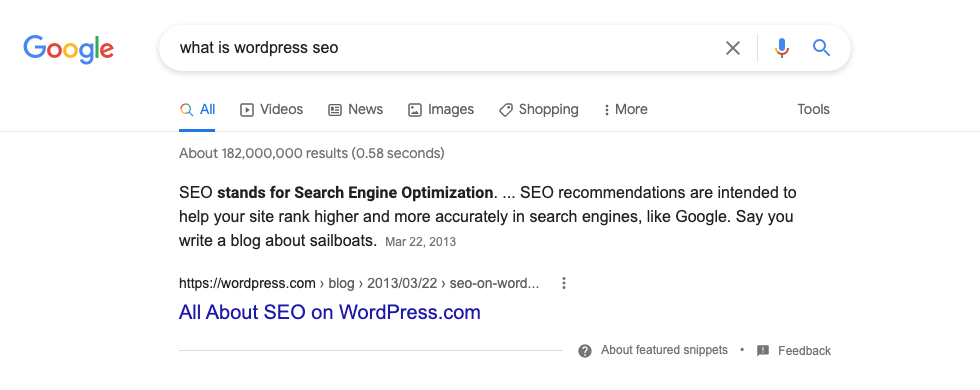Displayed on the screen is a Google search results page. Positioned at the top left corner is the iconic Google logo, featuring a vibrant color scheme: the "G" in blue, followed by letters in red, yellow, blue, green, and red. To the right of the logo, inside the search bar, the query reads, "What is WordPress SEO?". Immediately below, a horizontal menu highlights various search categories, with "All" emphasized in blue, followed by options for "Videos," "News," "Images," "Shopping," "More," and "Tools."

Underneath this menu bar, a summary line states that there are "About 182 million search results (0.58 seconds)". The image's main section shows the initial search results on a stark white background. The top result, written in black text, defines SEO with the phrase, "SEO stands for Search Engine Optimization." This detailed depiction offers a clear view of a Google search interface and the results provided for the query about WordPress SEO.